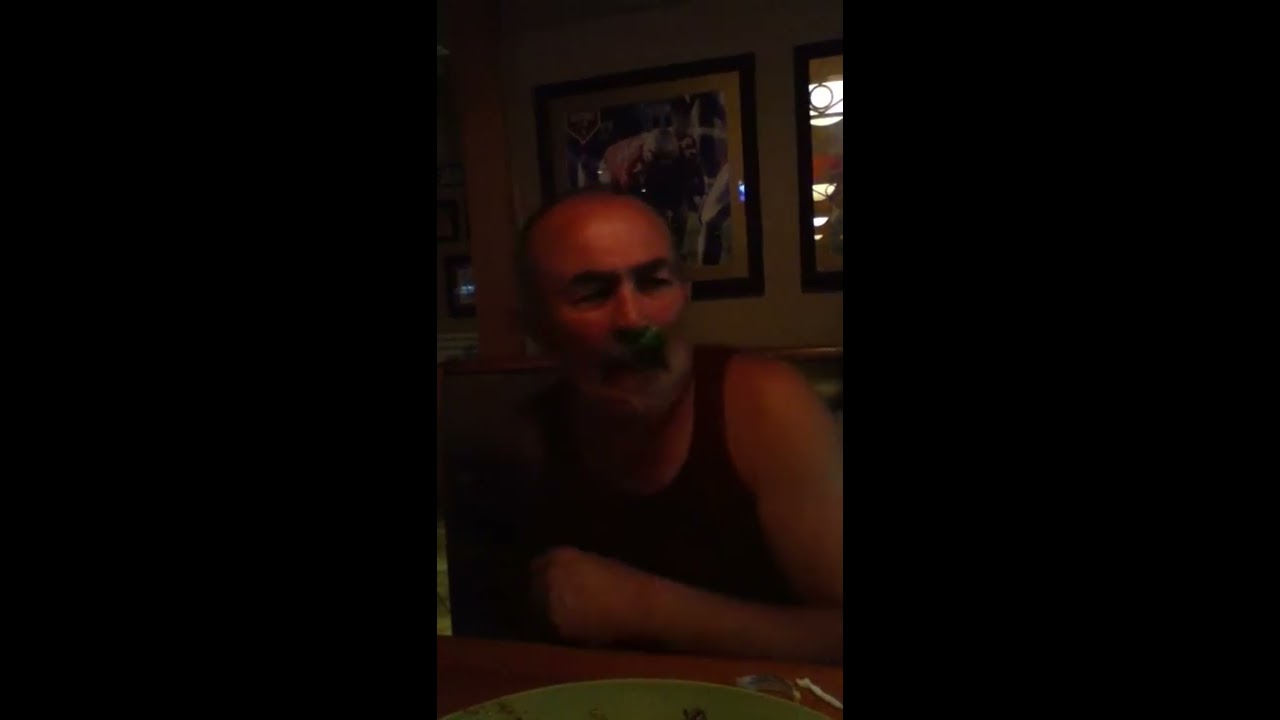In this slightly blurry and dark cell phone photo, a middle-aged man with a receding hairline and dark mustache is sitting at a brown table. He is wearing a black tank top and has a medium skin tone. His facial expression is somewhat angry, with eyes partially closed and lips slightly pulled down. One of his arms is bent at the elbow, resting on the table with his hand visible. On the table in front of him is a green plate and two indistinct objects that might be silverware. The plate appears to be pushed away, and its contents are unclear. The room around him is dimly lit, making details difficult to discern. Behind him, the beige wall features multiple framed pictures and what appears to be a window. The booth he is seated in is olive green with a wooden brown frame. Additionally, there is a large black border along the left and right sides of the image.